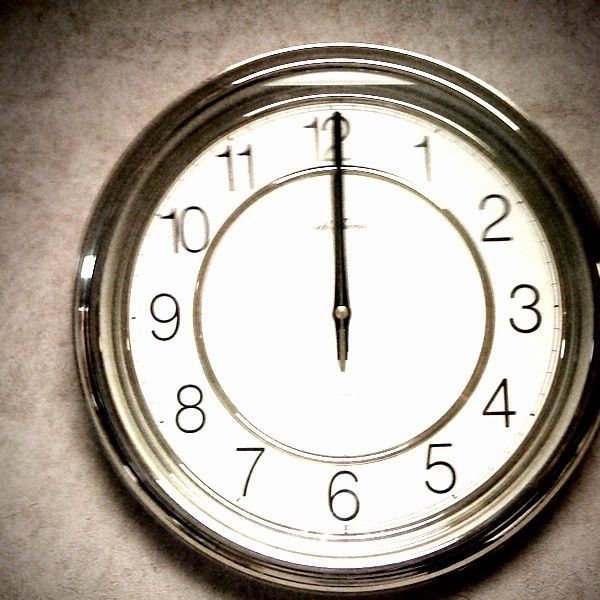In this square image, we are looking at a photograph of a wall featuring a distinctive faux finish paint job in shades of brown and tan. Mounted prominently on this wall is a round, gold-colored wall clock. The clock has gold numerals marking all twelve hours: 12, 1, 2, 3, 4, 5, 6, 7, 8, 9, 10, and 11. Notably, the clock only possesses one hand, the longer minute hand, which extends to reach the numbers. It is missing its second hand. A silver screw is visibly holding this lone hand at the center of the clock. Beneath the number 12, there is a name written in small script, likely indicating the brand of the clock, but it remains unreadable due to the blurriness of the photograph.